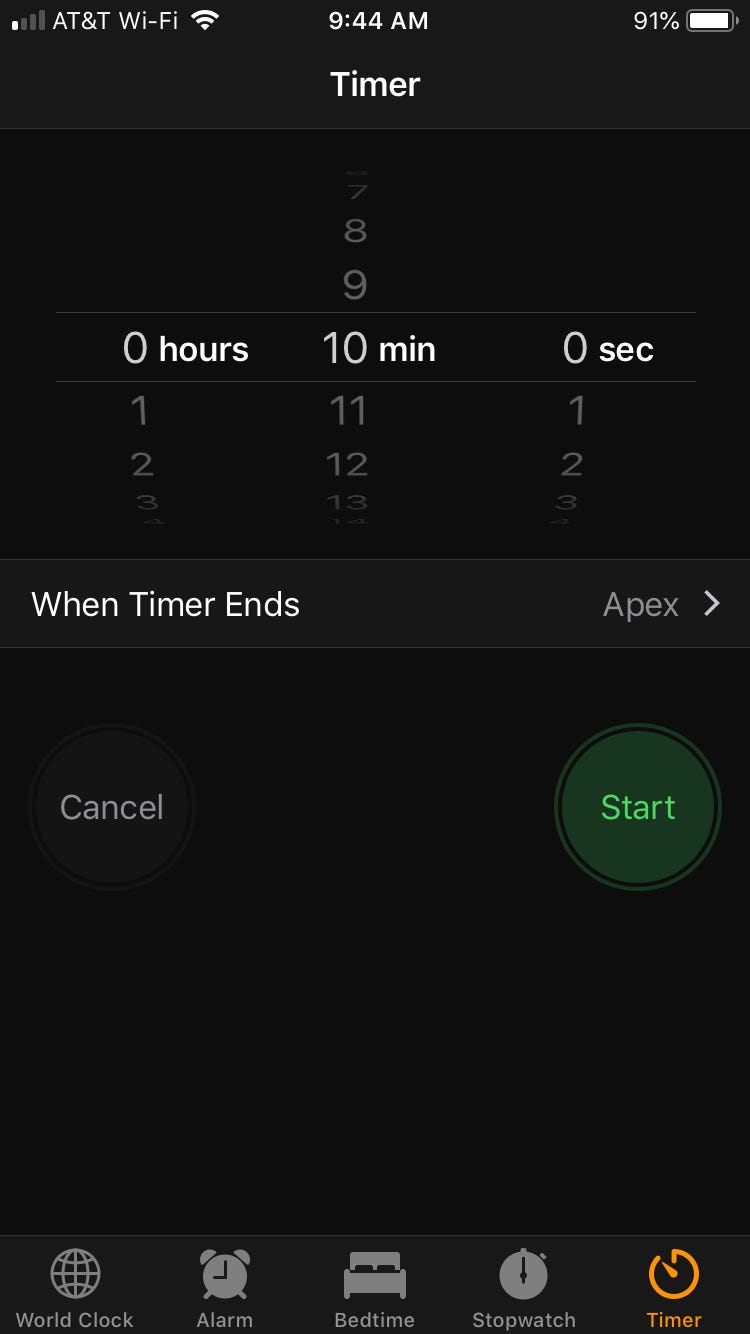The screenshot depicts a smartphone screen with a predominantly black background, divided into several distinct sections. At the very top, the status bar indicates the device's current wireless connectivity and battery status. Specifically, it shows one out of four bars for cellular signal strength, labeled as AT&T Wi-Fi with full Wi-Fi signal strength (three out of three bars), the current time of 9:44 AM in the center, and a battery charge level of 91% on the far right.

Directly below the status bar, a section is dedicated to timer settings. This area features three vertically scrollable columns of numbers that can be adjusted by touch, currently set to zero hours, ten minutes, and zero seconds.

Underneath these columns is a gray banner with white text that reads "When Timer Ends." To the left side of this banner is the word "Apex" alongside an arrow, suggesting the presence of additional options or settings that can be revealed by tapping.

Following the banner, a large black area contains two circular buttons. The left button is gray and labeled "Cancel," indicating it is not currently selected. The right button is green and highlighted with the word "Start" in light green, signaling it is the active selection.

At the very bottom of the screen, five navigation options are displayed: World Clock, Alarm, Bedtime, Stopwatch, and Timer. The Timer option is currently selected and highlighted in orange.

This detailed interface suggests the user is setting a timer on their smartphone, currently configured for ten minutes, and ready to initiate by pressing the "Start" button.